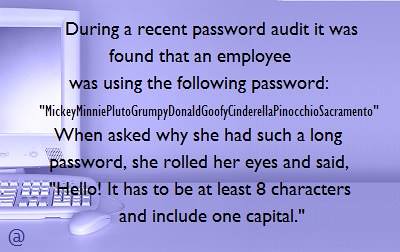This humorous image is a meme featuring black text over a light purple background, accompanied by an illustration of a vintage desktop computer, including the monitor, keyboard, and mouse on the left-hand side. The bold text reads, "During a recent password audit, it was found that an employee was using the password: 'Mickey, Minnie, Pluto, Grumpy, Donald, Goofy, Cinderella, Pinocchio, Sacramento'." When questioned about her extended password, the employee rolled her eyes and replied, "Hello, it has to be at least eight characters and include one capital." The meme humorously highlights the literal interpretation of password requirements using a series of capitalized Disney character names and a city. An additional detail at the bottom of the image is an "@" symbol, adding to the digital theme of the joke shared widely online.